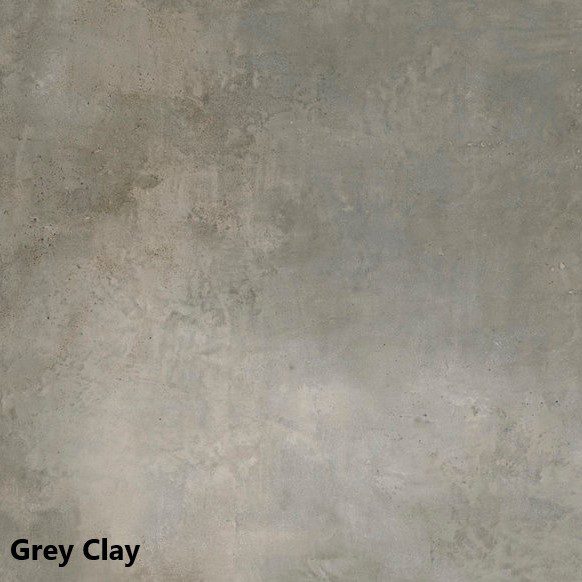The image features a highly detailed painting that primarily resembles a rough, textured gray wall. The surface, slightly varied with shades of gray, white, beige, and touches of brown, gives a realistic impression of old stone or concrete, mimicking a basement or industrial setting. The predominantly gray area is uneven, presenting a pattern of meandering textures that indicate wear and age. In the bottom left corner, in black typeface, the words "gray clay" are clearly inscribed, standing out against the monochromatic background. The overall piece is symmetrical, focusing on the extensive gray surface which encompasses the entirety of the image.